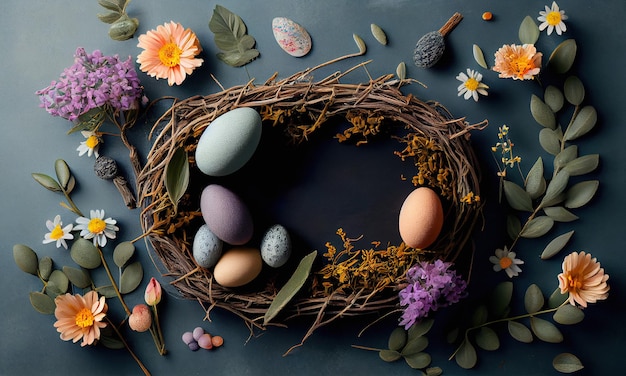The photograph captures an exquisitely detailed, oval-shaped wooden wreath made from interlocking brown sticks, showcasing a high level of artistic skill. The wreath, reminiscent of a bird's nest, serves as a canvas for an array of elements laid out in an aesthetically pleasing manner. Inside the wreath, there are various eggs of different sizes and colors, including orange, blue, gray, purple, and speckled varieties, with two of the smaller eggs notably having spots. Surrounding the wreath are clusters of artificial flowers and leaves, featuring hues such as purple, orange, peach with yellow centers, and pink, alongside some lavender and orange daisies. Yellow leaves and a pinecone add to the natural yet whimsical theme. Additional decorative elements such as pebbles and seeds are arranged around the wreath, all set against a striking dark teal blue background. This carefully composed arrangement of materials suggests the image could be part of a tutorial for crafting a spring or Easter-themed wreath, making it a delightful and charming piece suitable for sprucing up any home during the spring season. The light source from the left-hand side casts intense shadows, enhancing the depth and texture of the composition.